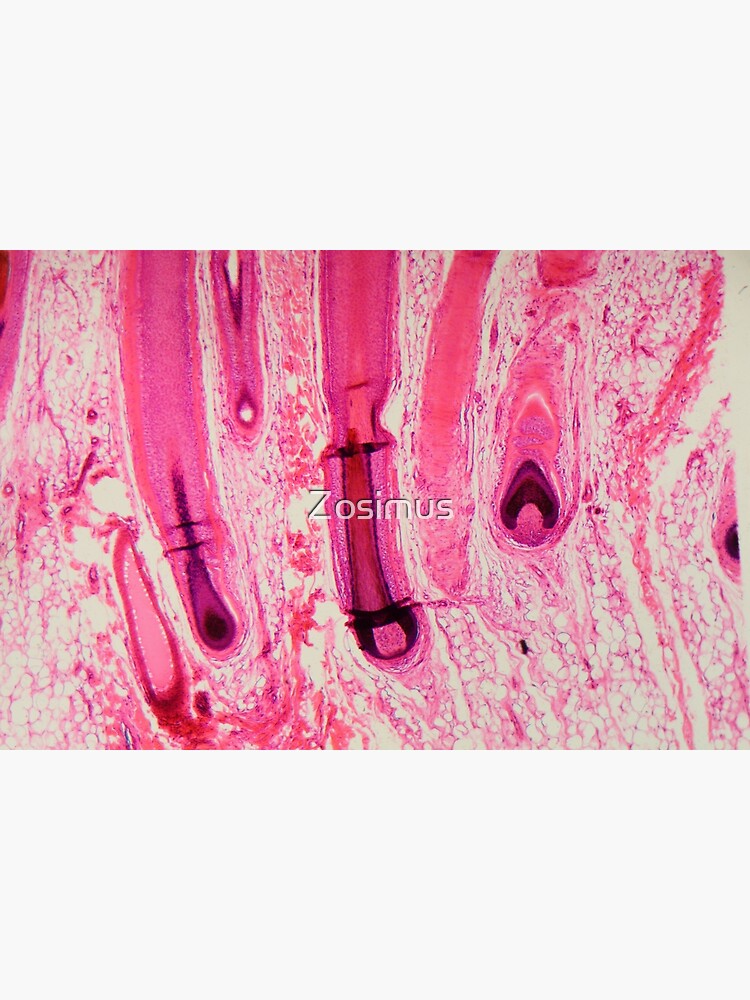This image features a painting centered on the canvas, with an intricate and detailed composition evoking the microscopic world seen under a slide. The painting is predominantly various shades of pink, ranging from light pink to burgundy and purples, over a light gray to white background. The main imagery includes long, tubular structures resembling hair follicles or cellular strands, descending from the top. Two principal strands, one slightly larger and more bulbous, extend downward, their bases forming shapes akin to avocados with black strings emanating from them. The positioning of these structures in the middle gives the appearance of organized chaos, accentuated by smaller similar forms and sporadic white circles that resemble bubbles. Adding another layer of complexity, there is a watermark in white text across the painting that reads "Zosimas." The overall look is that of an abstract, vibrant cellular or microscopic painting, blending elements of scientific illustration with artistic interpretation.